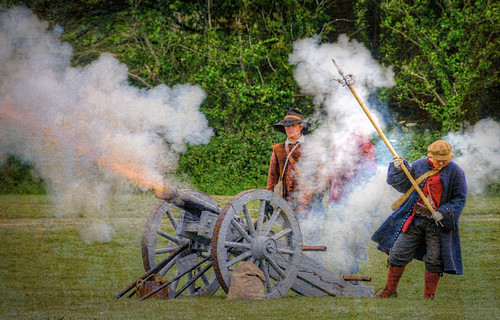In this small and grainy outdoor photograph, approximately three inches wide by two inches high, we see a captivating scene that appears to be a historical reenactment, potentially of the Civil War era. The image is set on a lush, green grass field, which occupies the bottom half of the photo, while the top half is adorned with thick, bushy foliage. At the center forefront stands a vintage Old World-style cannon with its two large, spoked wooden wheels reinforced by brown metal bands. The cannon is aimed upward towards the left, and it's mid-firing, producing a vivid reddish-orange flash from its muzzle, surrounded by billowing white smoke, which also emits from the back end of the cannon.

Three figures are discernible amidst the smoke. The man on the left, who appears Caucasian, wears a black floppy hat and a brown top, his visage slightly obscured by the haze. To the right, another man sports a floppy brown hat, a red waistcoat, and a substantial blue coat, open in the center and adorned with numerous buttons. He holds a long wooden staff, likely used for loading the cannon. Both men are dressed in attire reminiscent of a historical military uniform, lending credence to the idea of them participating in a reenactment. A third individual is faintly visible behind a veil of smoke, his attire indistinct.

The scene is dynamic and vivid, capturing the moment of the cannon's discharge with striking detail against the serene outdoor backdrop.